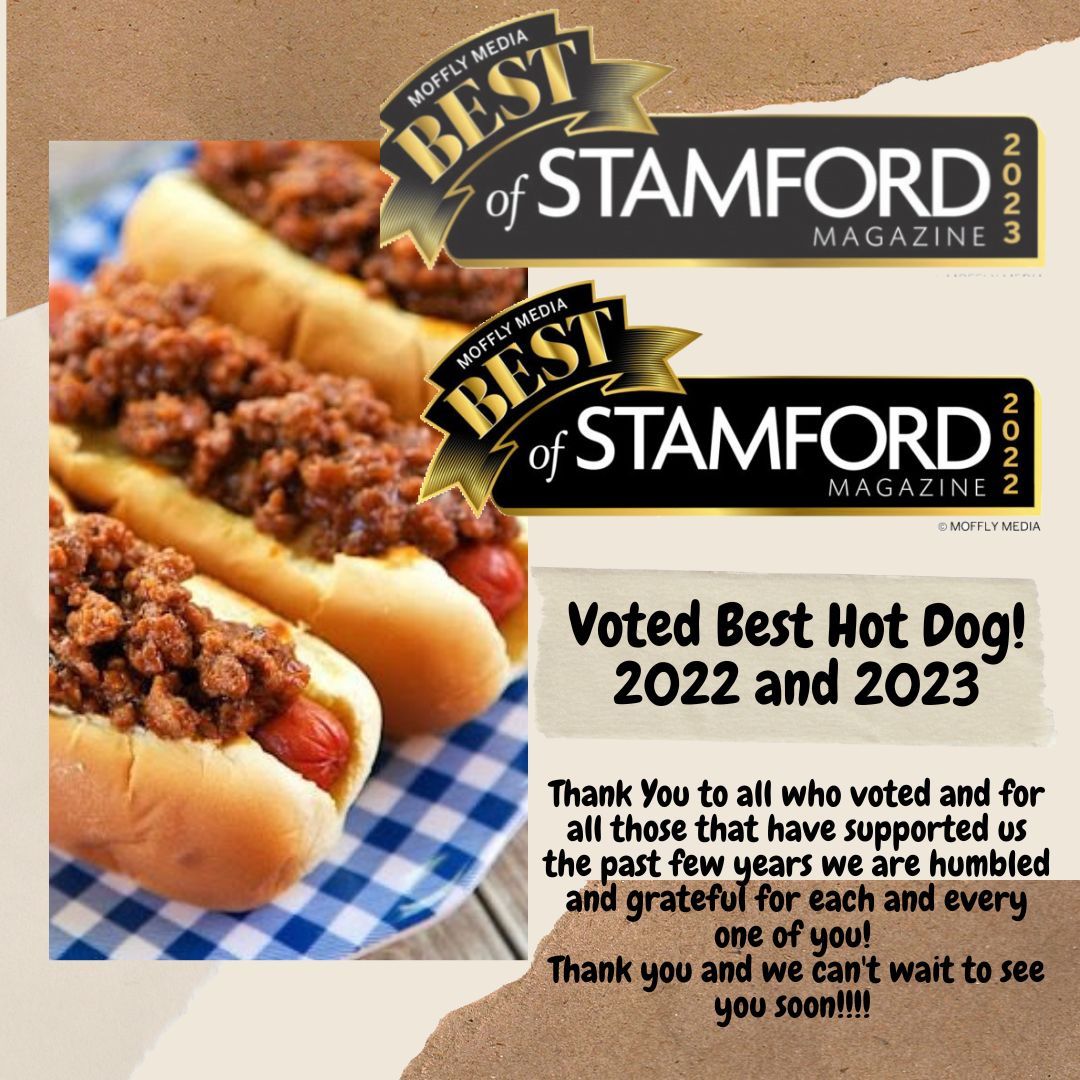In this color photograph with a portrait orientation, there is a vivid and appetizing ad for a hot dog restaurant. Dominating the left side of the image, three plump hot dogs are arranged side-by-side on a blue and white checkered cloth. The buns are neatly aligned, with savory brown chili generously piled on top, allowing a glimpse of the wiener at the right edge of each bun. The hot dogs are angled from the top left to the bottom right, with the central one fully visible and the outer two partially cut off.

On the right side of the image, a detailed banner is featured, showcasing the restaurant's accolades. At the top, the banner reads "Moffly Media" followed by "Best of Stamford Magazine" in a sleek design. There are two versions: one indicating the award for 2023 and another for 2022. The text "Voted Best Hot Dog 2022 and 2023" is prominently displayed in black. Below this, a heartfelt message in smaller black text thanks the customers for their support over the years, expressing the restaurant's gratitude and excitement to see them soon. The message ends enthusiastically with four exclamation points. The background behind the text is a brown and cream diagonal wavy pattern, contrasting beautifully with the vibrant colors of the food and the clean design of the text elements. This image perfectly blends photographic realism with graphic design, creating an engaging and mouth-watering advertisement.